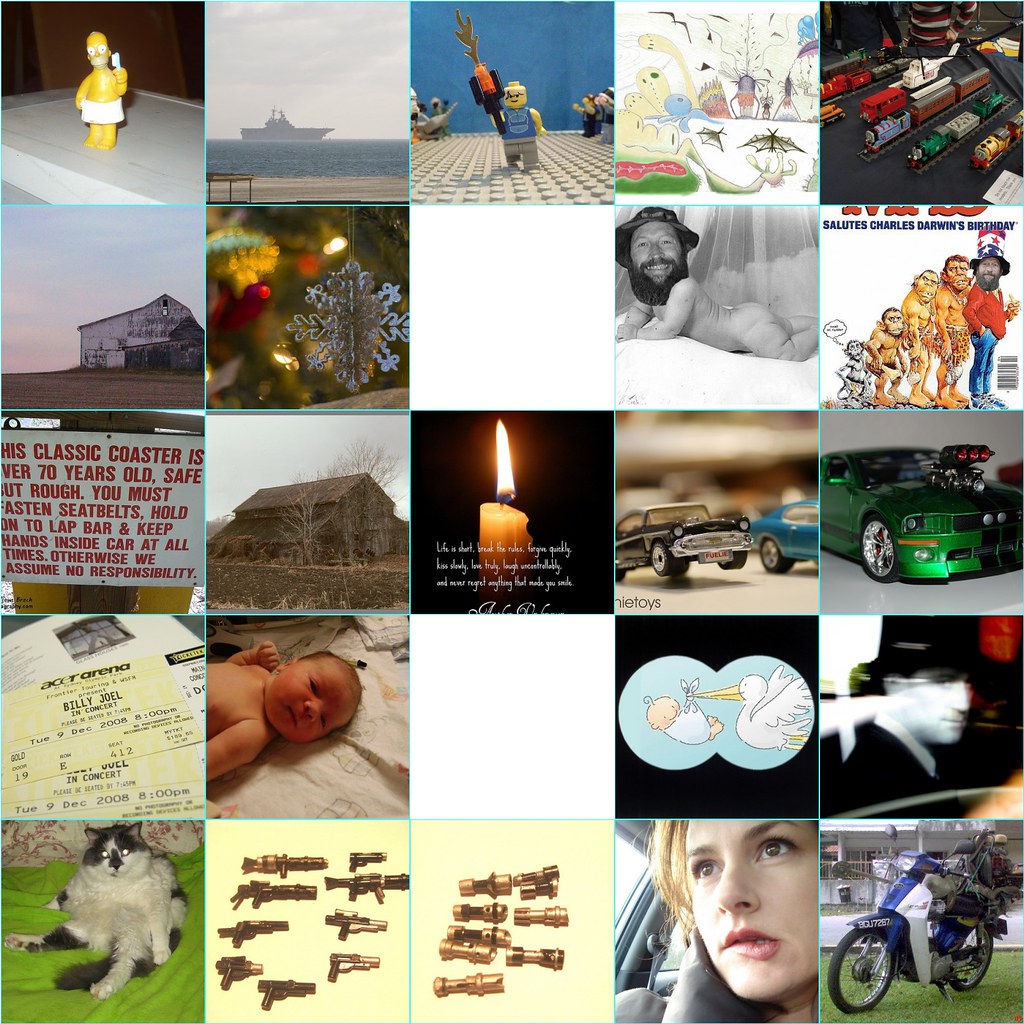The image displays a vibrant collage composed of 25 square photos arranged in a five-by-five grid. This visual compilation features an eclectic mix of subjects, including a Bart Simpson figurine, a Lego figure, and a large ship on the water. Amongst these diverse images, there are also pictures of a candle, a race car, and a Hot Wheels toy car. A baby, a motorcycle, and a woman sitting in a car also feature prominently. The grid further includes photos of guns, a cat, and Billy Joel concert tickets, adding layers of intrigue and personal interest.

Exploring the first row from left to right, one can see Homer Simpson, a ship on the horizon, a Lego figurine, a drawing of an alien, and a Thomas the Tank Engine train set. The second row starts with a barn, followed by a close-up of a Christmas decoration, a blank white box, an image of a man's face superimposed on a baby’s body, and a peculiar drawing of a figurine. Other notable images include an orange candle in the center, a man's bearded face, a green car, bullets, a woman's face, a sign in red print, an old house in the background, and myriad other elements, all amalgamated in a checkerboard pattern to create a complex and visually stimulating montage.